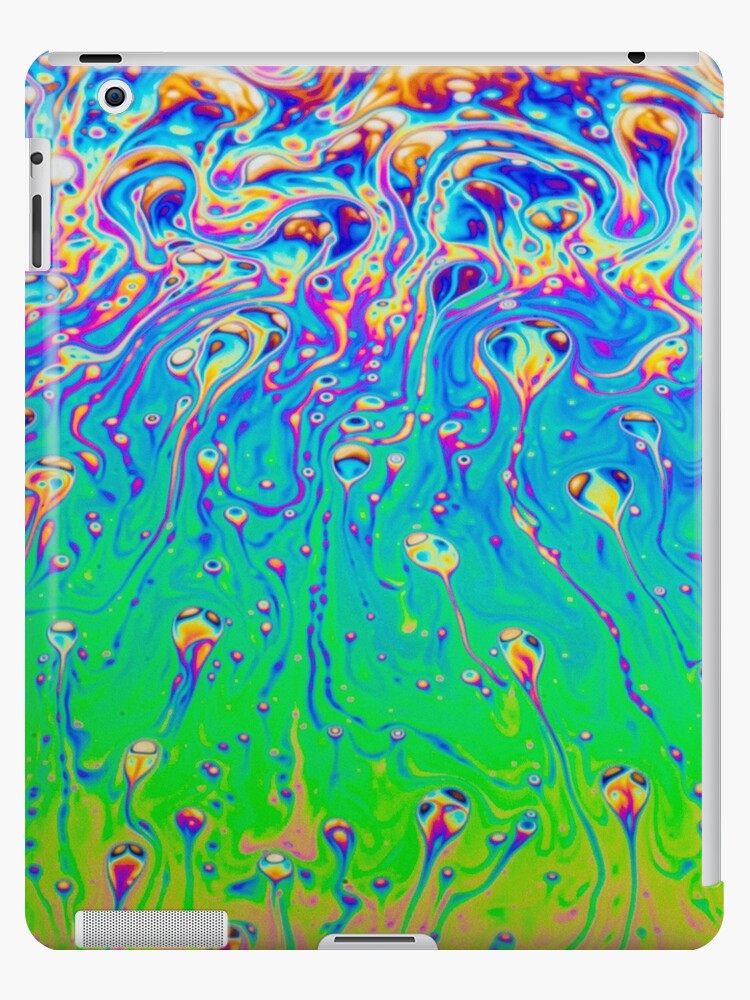The image depicts an abstract, psychedelic phone or tablet case viewed from the back. The top section features swirling, bubble-like patterns in shades of blue, brown, and purple that resemble raindrops merging into a water-like surface. As you move down, the colors transition through green, yellow, and blue, with various hues of blue, yellow, and purple raindrops continuing the vibrant, mixed descent. From the bottom upwards, the colors shift dramatically from yellow to green, blue, purple, and even reddish tones, with intricate, bulbous strand patterns in yellow, purple, and touches of orange and dark purple adding to the elaborate design. Functional details are also visible: a port at the bottom, a speaker port on the left side, a headphone jack and a sleep mode button on the upper left, and volume buttons—printed in white—on the side and top corners.